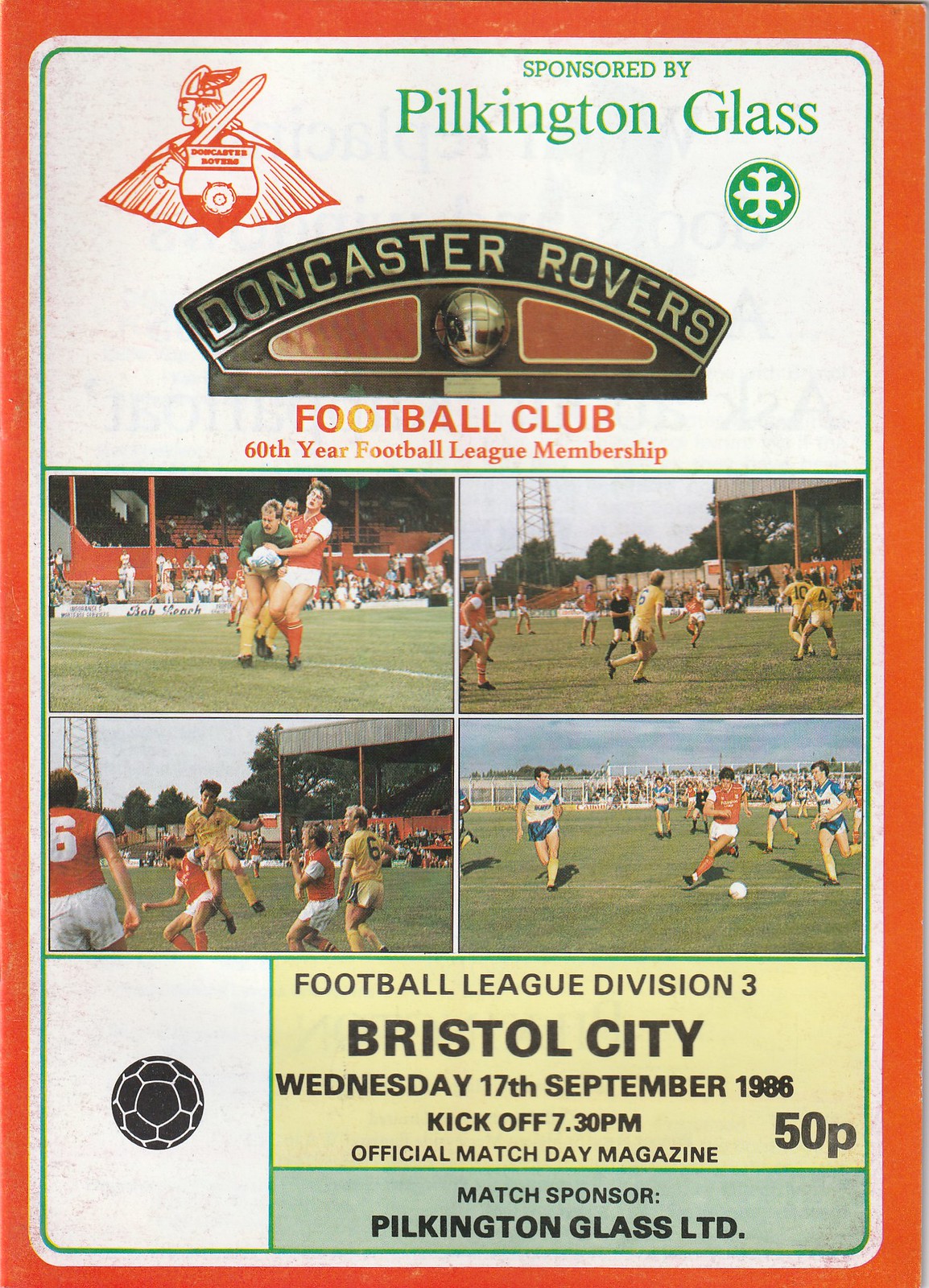The cover of the soccer program features a prominent orange border with a white center. At the top, in green text, it states "Sponsored by Pilkington Glass Limited." The upper left corner showcases a drawing of a Viking with a sword, signifying the Doncaster Rovers Football Club. Below this, it reads "Doncaster Rovers Football Club, 60th Year Football League Membership." The central portion of the cover contains a 2x2 grid of four equally-sized images depicting various soccer games, with each image portraying teams in the midst of play. The lower third of the cover displays a black soccer ball next to a yellow banner with the text: "Football League Division 3, Bristol City, Wednesday, 17th September 1986, Kickoff 7.30 p.m., Official Match Day Magazine 50p." Below this, in a green banner, it reiterates the match sponsor as "Pilkington Glass Limited."